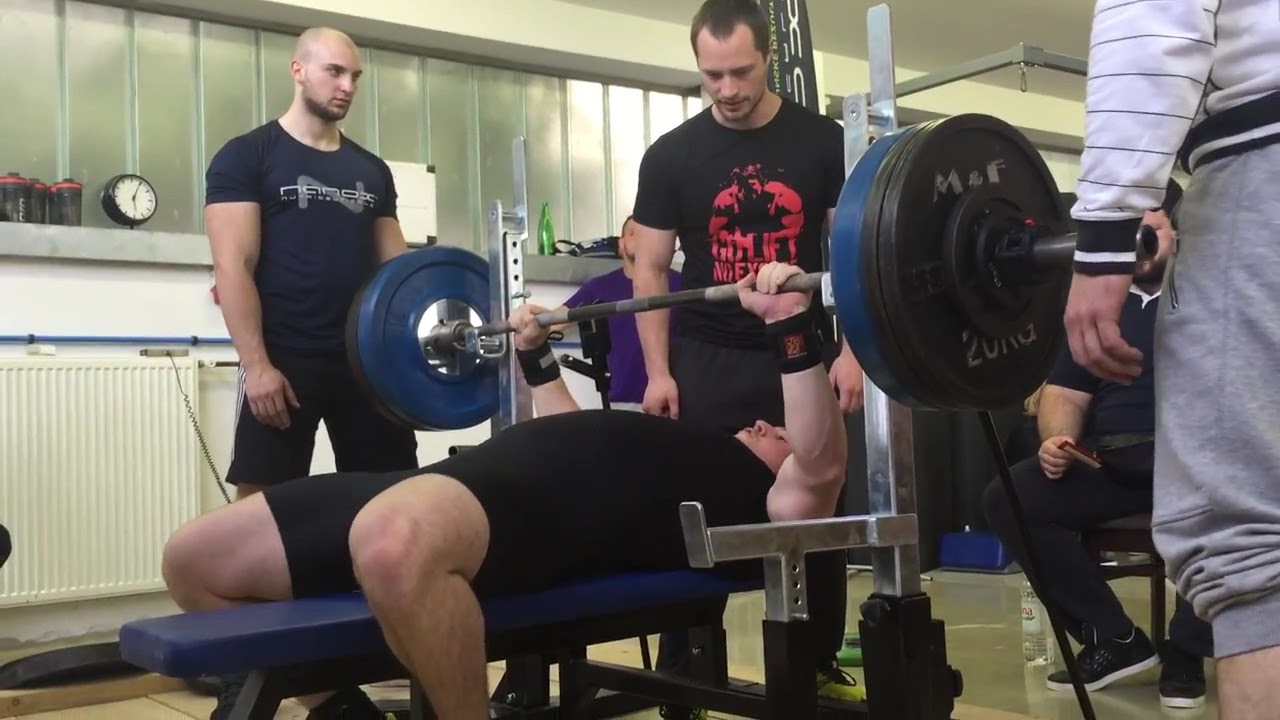In this detailed gym setting, a muscular man in a black shirt and black shorts is lying on a blue bench press, preparing to lift a heavily weighted barbell above his head. He wears black wrist supports, and his feet are firmly planted on the ground. Surrounding him are five or six individuals, all seemingly trainers or fellow gym-goers, attentively spotting and encouraging him. Notably, one spotter in a black shirt with red text stands at the center, offering close support. Another balding, bearded man in a blue shirt and black shorts stands to the left. In the background, a person in a purple shirt and another in black pants are visible, adding to the sense of communal effort. The gym features a white plaster ceiling, a glass wall, and rows of black and blue weight discs on metal rods, enhancing the atmosphere of focused physical training.